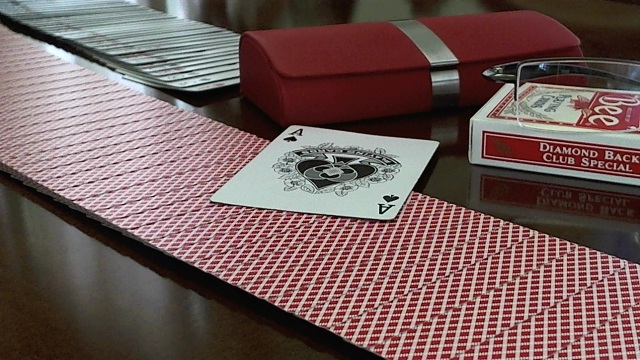This realistic photograph is a horizontal rectangle capturing an intimate close-up of a tabletop scene. The table surface, a shiny dark brown wood, serves as the backdrop. Positioned towards the top center of the image is a prominent red glasses case with a metal latch. To the right of the glasses case lies the box for the playing cards, distinctively white with red designs. The side of the box displays a red rectangle with the text "Diamondback Club Special" in white, while the top features another red rectangle with the letter "B" in white text. A pair of black-framed glasses rests atop this card box.

Dominating the image is a spread of horizontally stacked playing cards extending diagonally from the top left to the bottom right. These cards showcase a red background adorned with white crisscross stripes. Sitting prominently atop this cascade of cards is the Ace of Spades, face up, featuring its classic white design with a black spade and the letter "A". On the far left side of the image, a separate row of face-up cards with white backs appears, though their details remain indistinct. The overall composition captures a moment of casual organization, with each element carefully placed on the glossy tabletop.